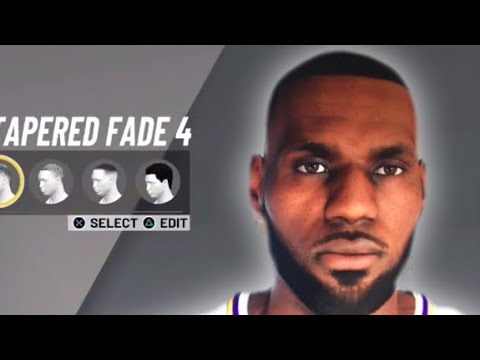In this image, we're in a character customization screen of a basketball video game, resembling the style of NBA 2K. The screen prominently features LeBron James, showcasing a highly detailed and close-up view of his face, which appears ready for any customization. The game interface allows players to modify various elements of LeBron’s appearance, focusing currently on his hairstyle. The displayed section is titled "Tapered Fade," and it provides different haircut options, with one such option closely mirroring LeBron’s current real-life hairstyle. It’s slightly unclear whether this is an actual in-game LeBron James model or an impressively accurate custom-created character.

The PlayStation interface is evident, indicated by familiar symbols and buttons, prompting players to select or edit further customization options. The background is decorated with abstract shapes and shades of gray, adding a modern, dynamic feel to the scene. Additionally, LeBron James is depicted with a subtle glow or halo effect around him, emphasizing his prominence in the display.